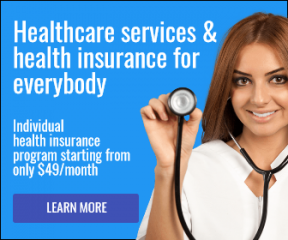This image, depicting healthcare services, features a square-shaped blue background with various design elements. In the top left corner, white text reads "Healthcare Services: Health Insurance for Everybody." Beneath this, additional text states, "Individual Health Insurance Program Starting From Only $49 a Month." Below the text is a rectangular button in a dark blue-purple color with the words "Learn More" in white.

To the right of the text, there is an image of a nurse. She has brown hair and dark black eyebrows, and she is smiling warmly. The nurse is wearing a white jacket or shirt and has a stethoscope around her neck, holding the end up as if preparing to use it for an examination. The overall impression is one of professionalism, warmth, and accessibility.